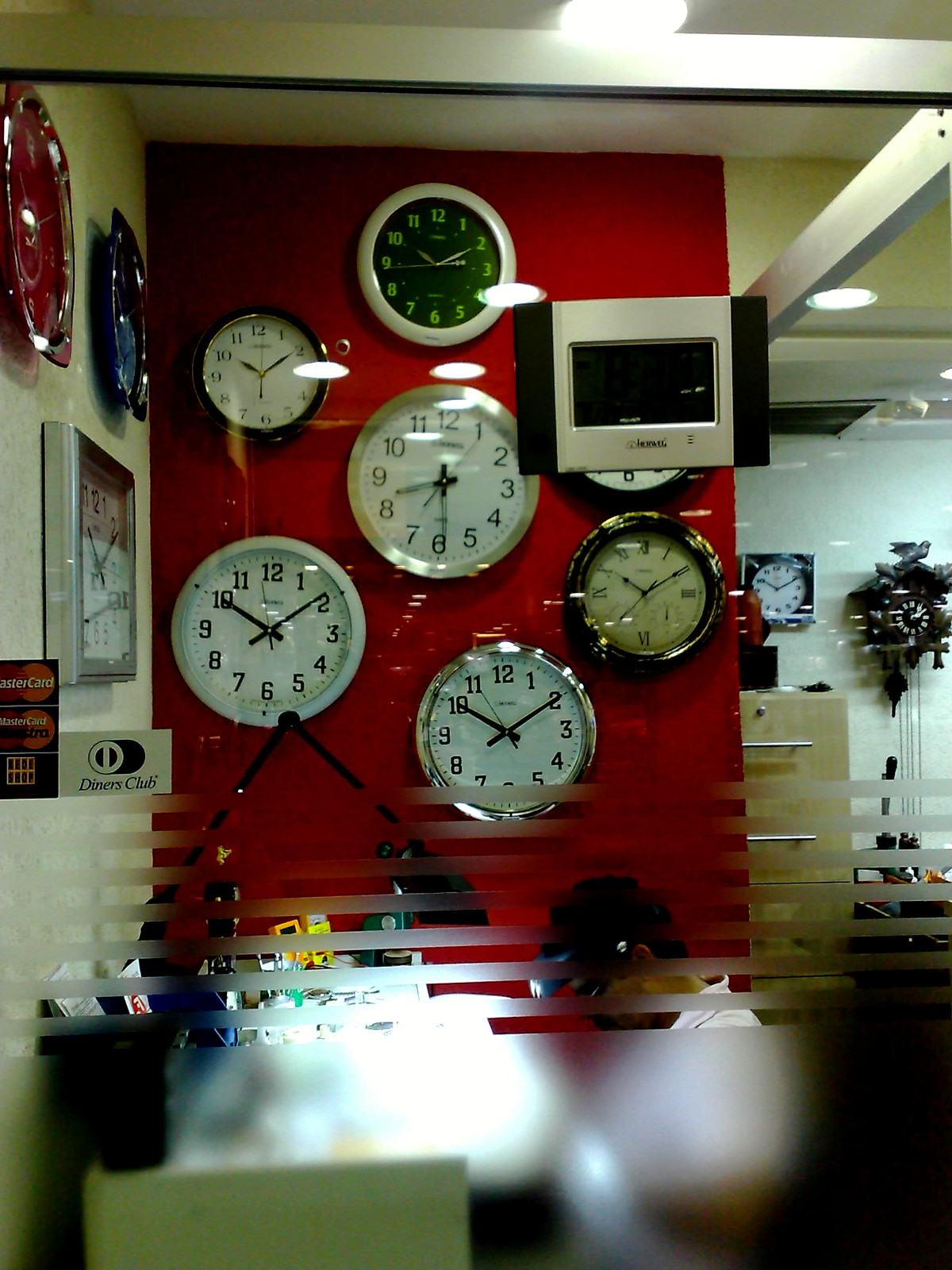A rectangular photograph captures a modern office setting, dominated by a large glass window in the foreground. The window features multiple stripes of frosted decoration, with the bottom section completely blurred out due to the frosted design. Through the glass, a small, rectangular white desk can be seen, occupied by an individual wearing jeweler's glasses resting atop their head, intensely focused on their work. Several logos are visible on the glass, including two rectangular ones that read "Mastercard" in white text and another that reads "Diner's Club." The background reveals multiple clocks mounted on the walls, emphasizing the international or time-sensitive nature of the office environment.